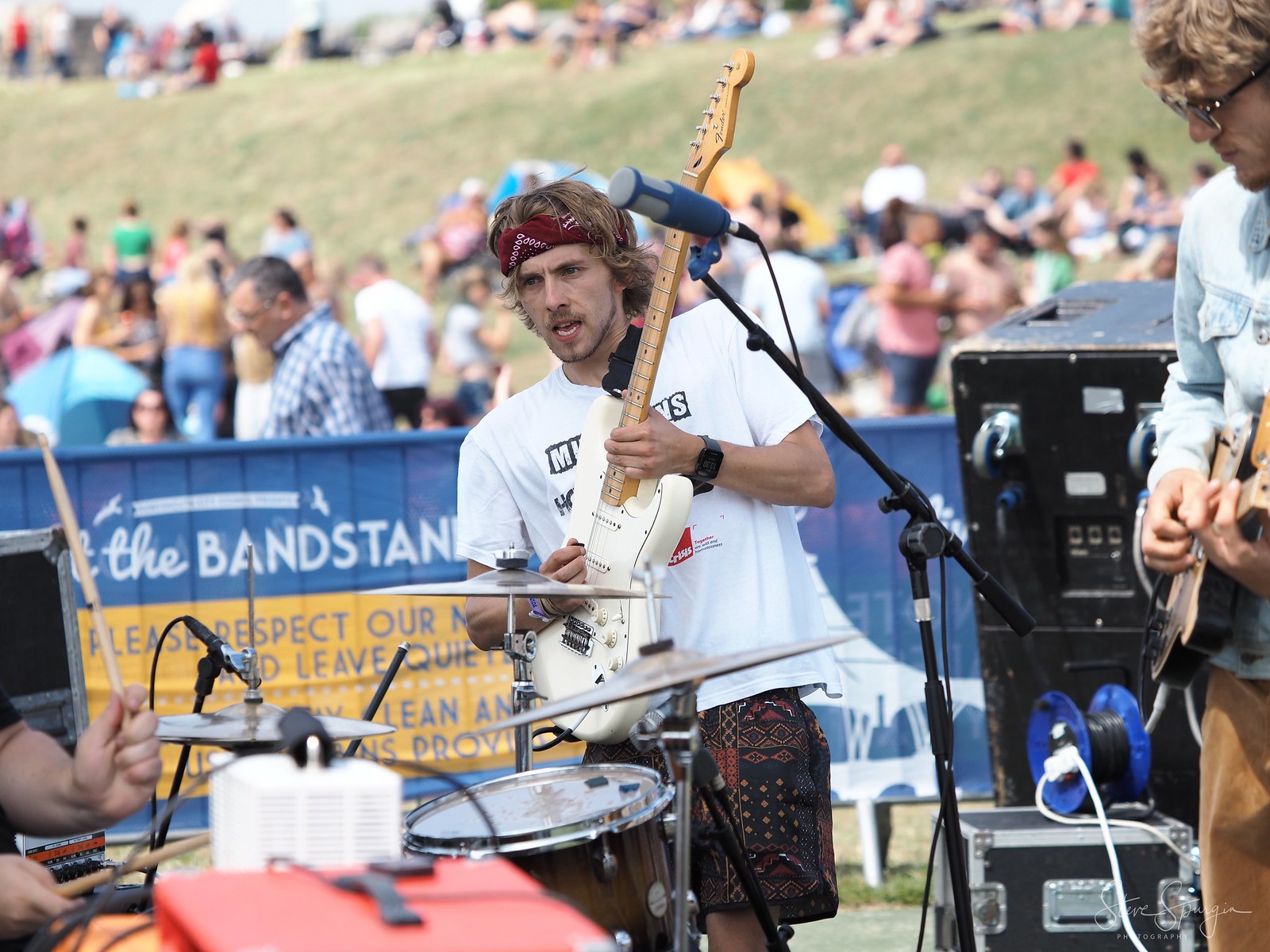In this vibrant, full-color photograph captured at a daytime outdoor concert, three musicians are performing with enthusiasm. Central to the image is a blonde or brown-haired man in a white t-shirt and patterned shorts, energetically strumming a white electric guitar, and wearing a red bandana that holds back his long hair. To his right, a man in a long-sleeved blue shirt and tan pants plays a bass guitar or another electric guitar, while the hands of a drummer, partially visible in the bottom left with a set of black drums, can also be seen holding drumsticks.

The scene unfolds in front of a striking backdrop; behind the band, there is a blue banner draped over a fence, with a crowd of concert-goers either standing or sitting on a grassy hill, adding a vibrant communal atmosphere. A sign reading "The Bandstand" asks attendees to "Please respect" and to "keep out of the artist's way." The photograph also captures various pieces of equipment, including a microphone, speaker, and wiring, all contributing to the authentic feel of a lively music festival on a fine day.